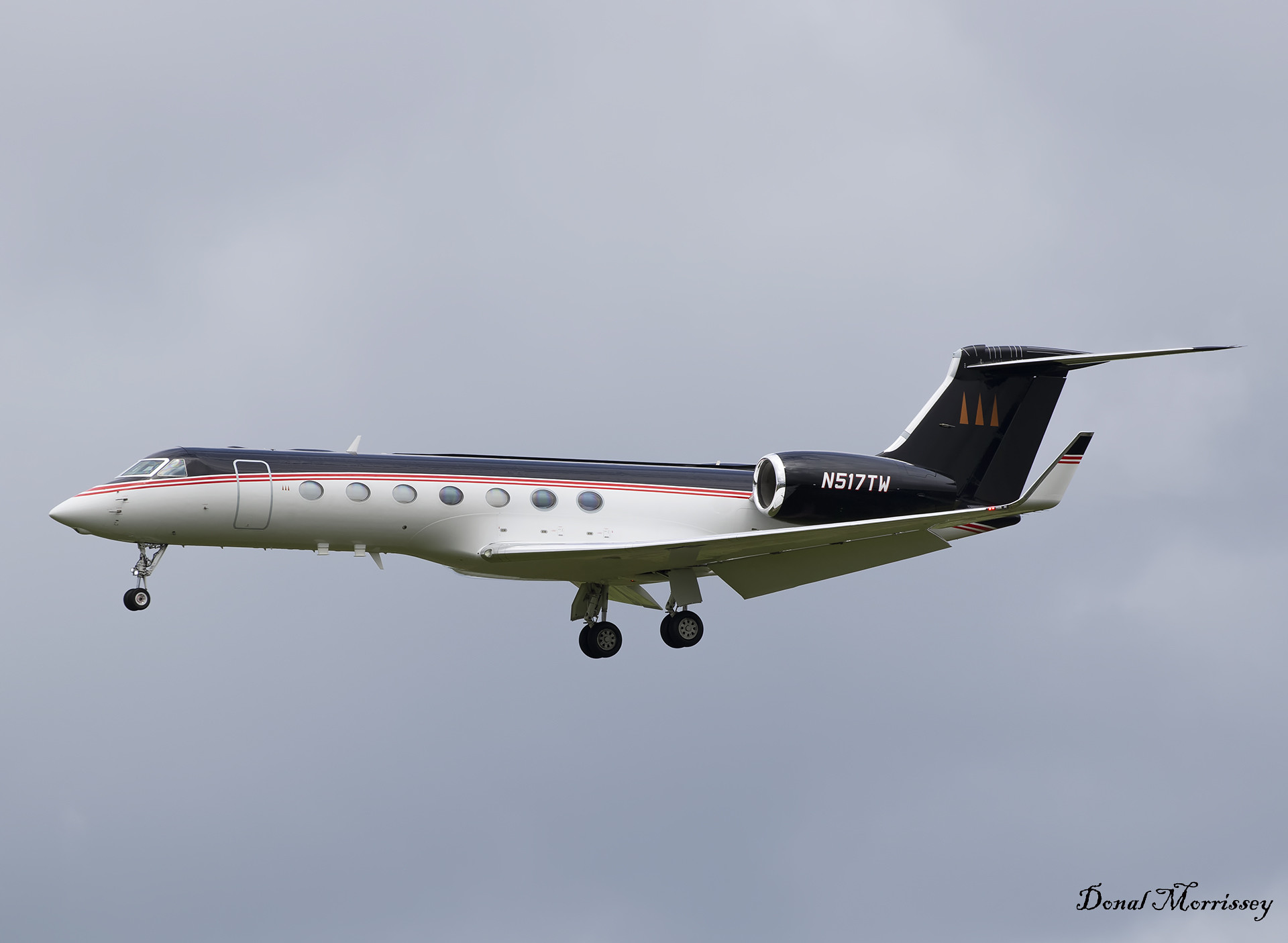The image depicts a white aircraft slightly left of center, flying from right to left, with its nose on the left side and tail on the right. The aircraft features a slimmer blue stripe on top and a couple of red stripes running horizontally from nose to tail underneath the blue. Below these red stripes, the main body is white, adorned with seven round windows. The engine on the visible left side is colored blue and displays the registration number N5177W in white. Further back, the tail is also blue, featuring some indiscernible gold design or lettering at the top. The aircraft's landing gear is extended, with two wheels visible in the middle and one under the nose. The backdrop is a uniformly gray, cloudy sky. In the bottom right corner of the image, "Donal Morrissey" is inscribed in small, black cursive text.